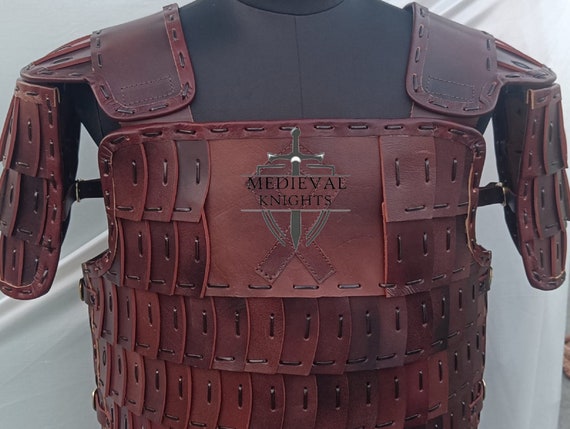This detailed photograph captures a close-up of a replica medieval armor suit, displayed on a black mannequin against a white backdrop. The armor, made of intricately tanned red leather or synthetic leather, includes a chest plate and shoulder plates meticulously assembled from multiple square pieces. These pieces are bound together by brass clasps and dark embroidery, creating a cohesive and historically evocative appearance. At the center of the chest plate, the words "Medieval Knights" are emblazoned in black, accompanied by a crest featuring a silver sword and two upward-extending objects. The well-lit setting highlights the craftsmanship and detailed leatherwork, making each element of the armor clearly visible.